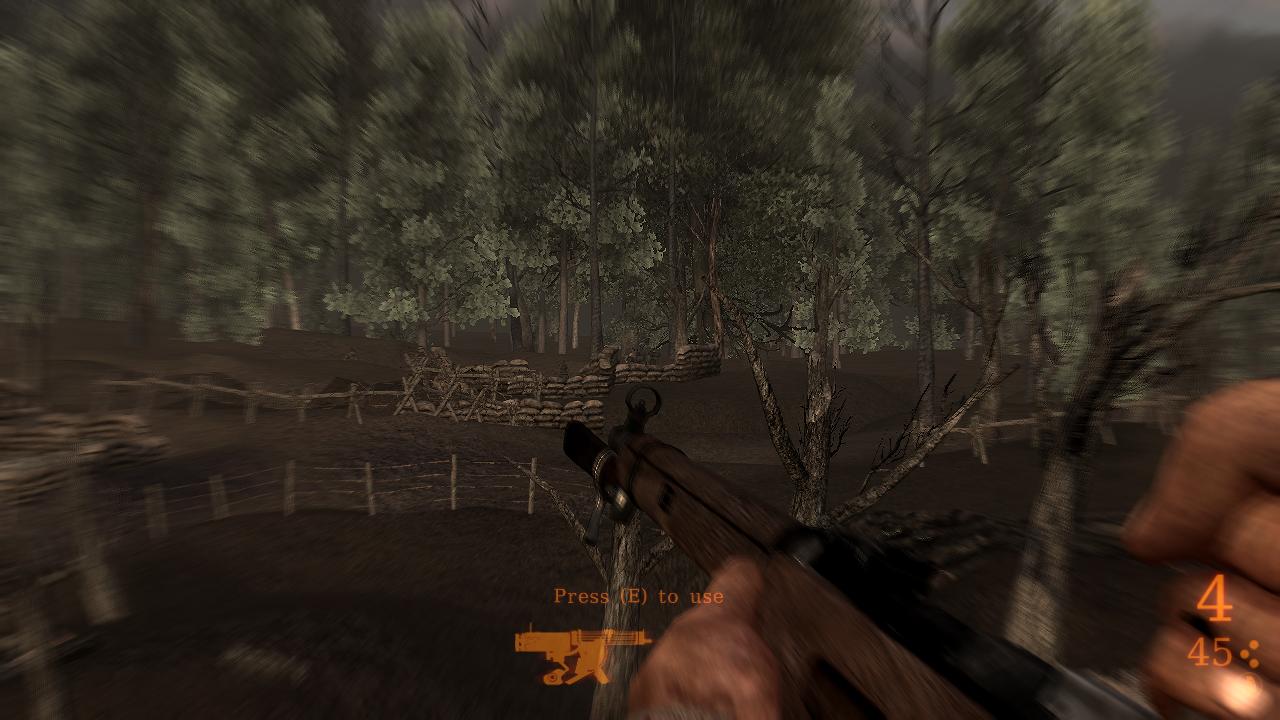The image captures a moment from a gameplay session, depicting a tense and atmospheric scene. In the lower section of the frame, the HUD displays critical information: an orange '4' followed by a '5', accompanied by three orange circles. Towards the center, a message in vibrant orange font reads “Press E to use,” indicating the interactive nature of the game. 

A character's hands, human and clad in tactical gloves, grip a rifle. The weapon features a detailed design with shades of black, brown, and silvery metallic elements. Surrounding this central focus, the game environment is revealed in moody, foreboding tones. Gloomy trees with brown trunks and dark green leaves populate the scene, contributing to the eerie ambiance. 

The backdrop includes a dilapidated fence, its brown slats appearing weathered and on the verge of collapse, further enhancing the atmosphere of decay. In the distance, sandbags are visible, hinting at previous or impending conflict, alongside dirt hills that form a rugged terrain. This richly detailed setting immerses the viewer in a post-apocalyptic or wartime landscape, emphasizing the gravity and intensity of the game.